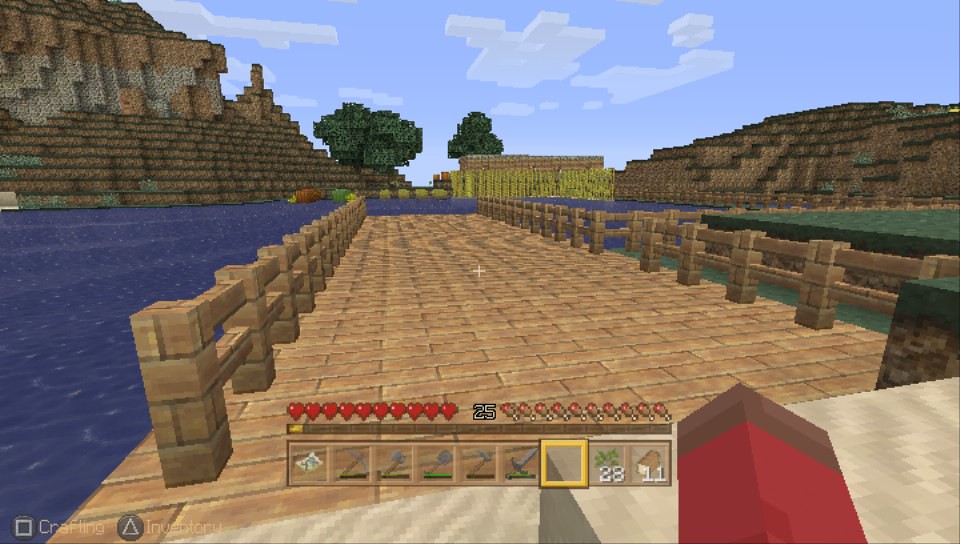The screenshot from the game Minecraft exhibits a quintessentially blocky, pixelated world. Central to the image is a long, tan tile pier or bridge extending over a body of blue water, bordered by a two-rail stone fence. In the background, the landscape features ambiguous, pixelated structures that resemble mountains, brown hills, green trees, or pyramids, evoking the aesthetic of a Lego-like environment. The foreground displays the player's interface, prominently showing their health with a line of red hearts and their hunger or other status indicators on the sides. At the center, there is a level indicator displaying '25'. Additionally, a yellow box signifies that the player possesses 28 units of a specific item, along with 11 units of lumber. The bottom interface includes options for 'Crafting' and 'Inventory,' accessible via the square and triangle buttons respectively, alongside icons for various weapons like swords and possibly hammers.